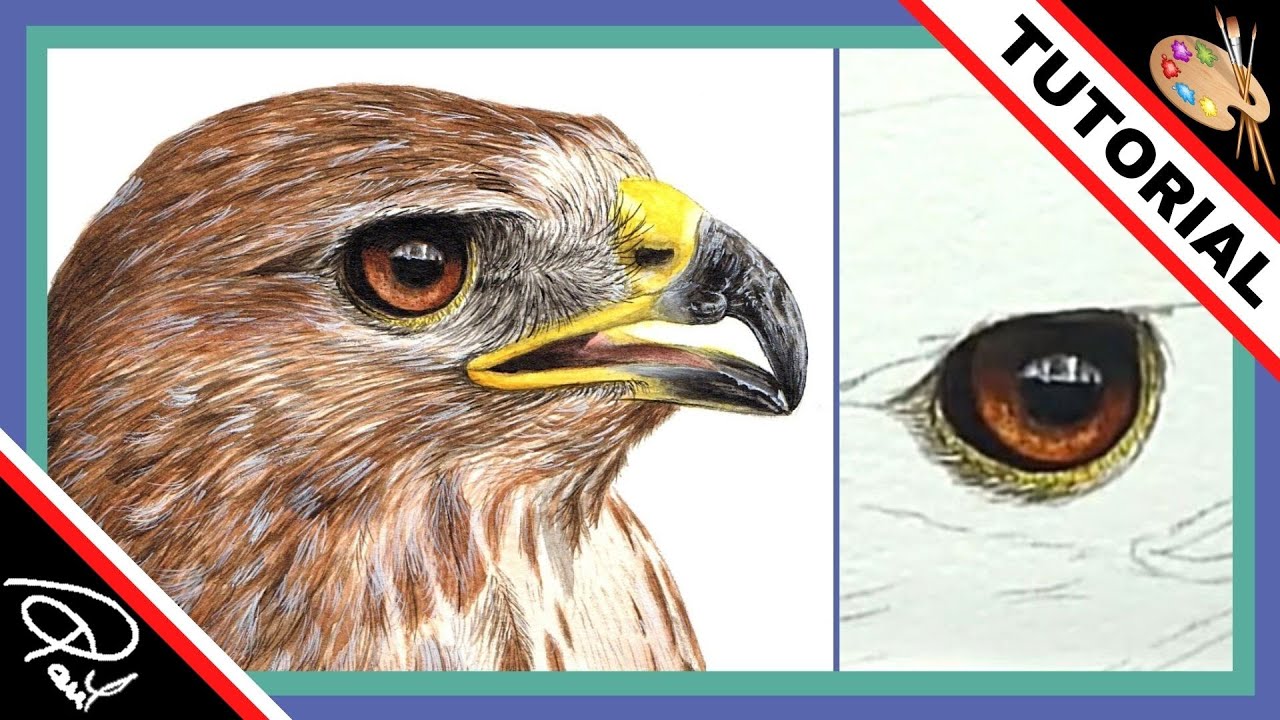This illustration features a detailed sketch of a bird, likely a bald eagle, situated on the left side of the image and facing toward the right. The bird is characterized by light brown feathers with gray tips, a black, rounded beak with a yellow edge near the mouth, and brown eyes. There is a close-up drawing of the bird’s eye, also brown, on the right-hand side. In the bottom left corner, the word "Paul" is written in white cursive lettering. The top right corner of the image displays a palette with various colors—green, purple, red, blue, and yellow—and some paintbrushes. This image is part of a tutorial, as indicated by the black capital letters "Tutorial" at the top, likely aiming to instruct viewers on how to draw the bird. The illustration is framed by green and blue borders, and the presence of the sketch and close-up detail suggests a step-by-step drawing tutorial format.